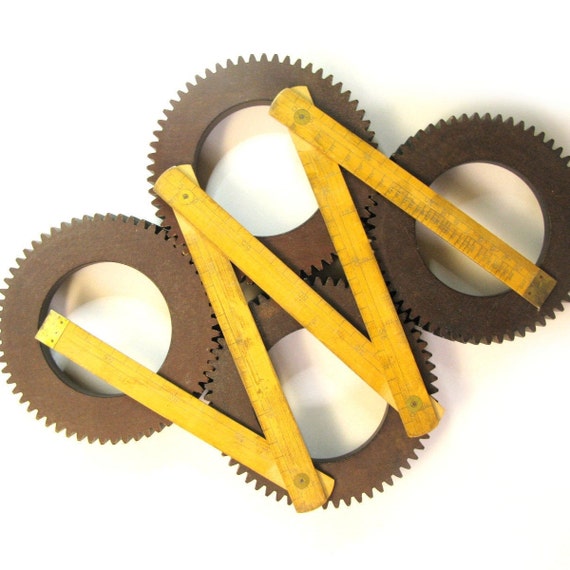The image depicts four similarly-sized, interconnected brown gears with serrated teeth made from a material that appears rusty. These gears are intricately arranged in an interlocking fashion on a white background, forming a cohesive W-shaped pattern diagonally. Overlapping the gears is an aged, foldable yellow measuring stick with faded markings, forming a zigzag arrangement due to partial retraction. You can also observe the shadows of the gears cast on the underlying surface, adding depth to the overall composition. The image captures a unique confluence of mechanical components and measuring tools against a stark, uncluttered backdrop.